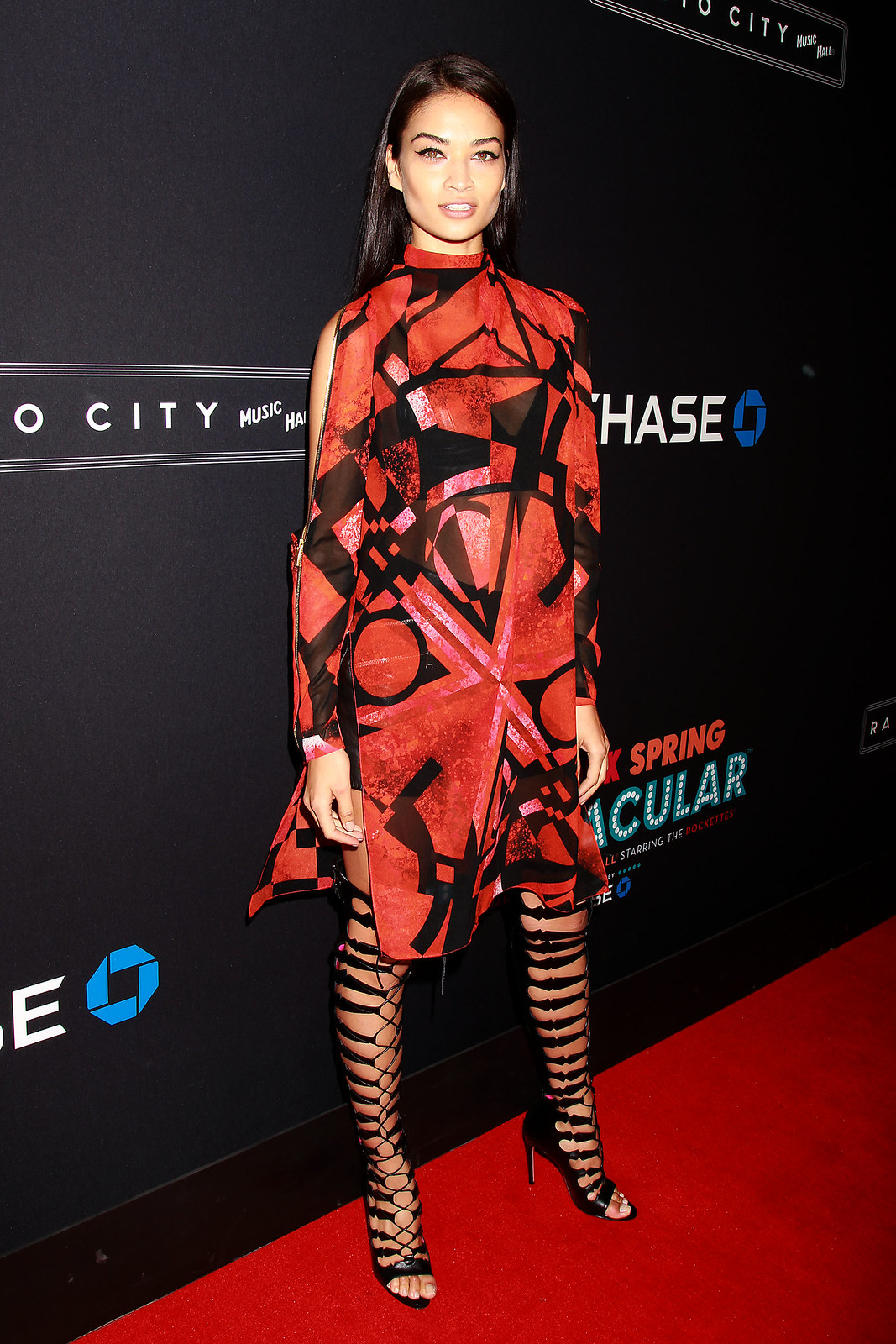In this striking image, an unknown actress or model, likely of Asian descent, graces a red carpet event with a radiant smile directed at the camera. She is adorned in a chic, modern, long-sleeved dress featuring a dynamic mix of black, red, and white triangles and circles that evoke modern art. Her high heels, designed with intricate straps that ascend to her knees, resemble knee-high boots with cutouts, showcasing meticulous stitches. Her long, shiny black hair cascades elegantly over her shoulders. The background is a black backdrop peppered with sponsor logos including Chase, Citibank, and Radio City Music Hall, with references to the Spring Spectacular Rockettes event. The overall scene captures both her fashionable attire and the glitz of a high-profile red carpet occasion.